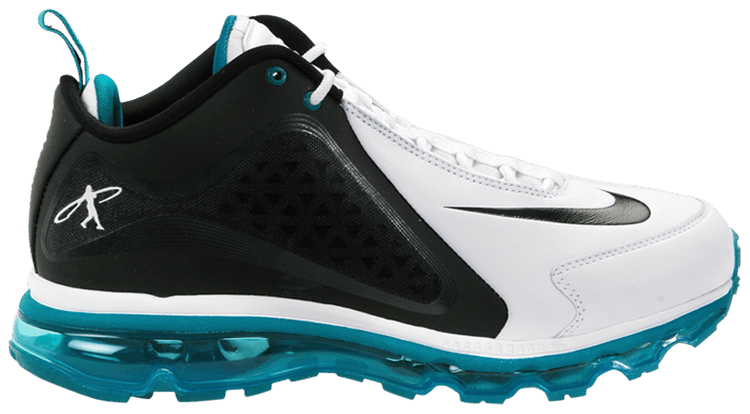This is a high-resolution, close-up stock photo of a Nike high-top athletic sneaker, designed for online shopping. The sneaker is set against a clean white background, highlighting its detailed features. The shoe predominantly features a striking black and white color scheme: the back half is black, transitioning seamlessly into white at the midsection and front. The toe cap is white leather with a prominent black Nike swoosh. The laces, made of durable white fabric, complement the shoe's sleek design.

The sturdy sole of the shoe is a transparent, rubberized teal aqua blue, extending into a distinctive, textured base that adds both style and functionality. This blue hue is echoed on the inner side of the tongue and the fabric loop at the heel, adding bursts of color to the monochrome body. The tongue itself is white, accented with blue detailing.

A unique feature of the shoe is a small emblem on the outer side, which depicts a silhouetted figure in white holding what appears to be a lasso, framed by a circular design. This detailed branding adds a playful yet sophisticated touch to the classic Nike aesthetic. The back of the shoe is structured with a fabric material, contributing to its hybrid style that merges elements of traditional tennis shoes with high-top sneakers.